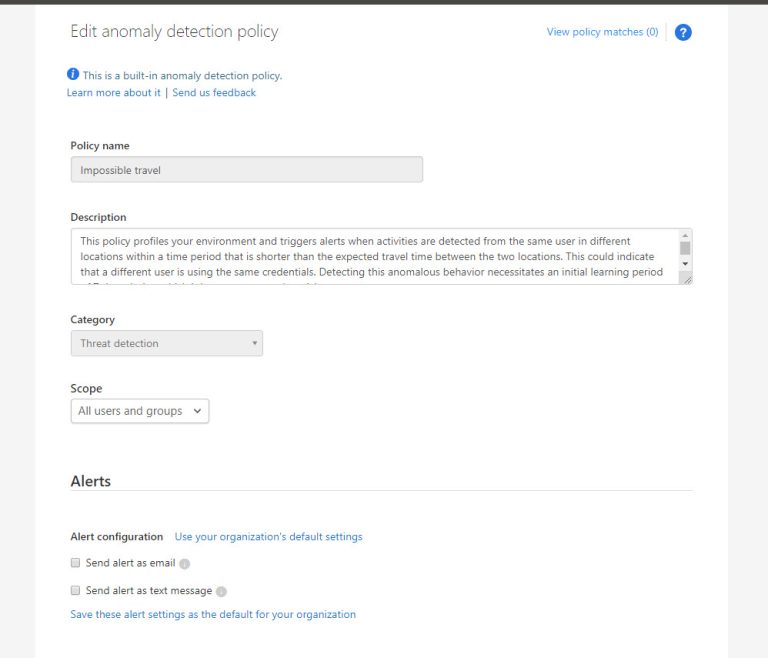The image displays a webpage titled "Edit Anomaly Detection Policy," showcasing an interface designed to configure a built-in policy for anomaly detection. The primary policy featured is named "Impossible Travel." This policy generates alerts when a single user's activities are detected from different geographical locations, indicating potential unauthorized access or compromised accounts.

At the top of the page, there are two hyperlinks: "Learn more about it" and "Send us feedback," providing additional resources and a way to contact support. Below these links, users can modify various settings such as the policy name and read its detailed description. The policy belongs to the "Threat Detection" category and is applicable to all users and groups within the organization.

Towards the bottom, the "Alert Configuration" section offers options for how alerts should be sent. Administrators can choose to use default organization settings or customize alert preferences with options to send alerts via email or text message.

The background of the webpage is white, and the text is displayed in a black font, ensuring clear visibility and readability. The overall interface appears to be aimed at network administrators or security professionals tasked with monitoring and responding to potential security threats by detecting anomalies in user behavior.